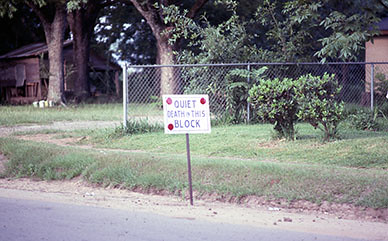The image depicts a residential street scene framed in landscape mode, with a noticeable and somewhat ominous sign at its center. The sign is mounted on a brown pole and reads, "QUIET, DEATH IN THIS BLOCK," in blue capital letters. It is a square, white sign featuring three large red dots positioned in the top left, top right, and bottom left corners. The sign stands along the edge of a grassy verge that is about a foot higher than the adjacent road, which appears to be a minor side street rather than a main road.

To the right of the image is a chain-link fence, behind which are numerous trees and bushes. Elevated terrain leads to private properties suggesting a residential area. A dilapidated wooden house or cabin is visible in the upper left corner, partially obscured by two thick tree trunks, with a wooden chair placed on its porch. In front of the house, near the trees, lie some white blocks. Extending across the background, there are more bushes and trees adding to the greenery. The overall scene suggests a quiet, perhaps rural, neighborhood setting, potentially in the United States. The combination of the sign’s message and the serene residential backdrop creates a striking and unusual contrast.